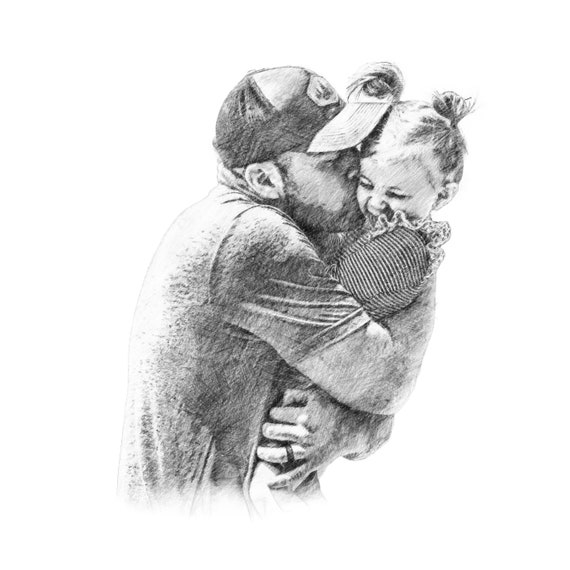This black and white pencil sketch intricately depicts a younger to middle-aged man joyfully embracing and kissing a little girl, approximately three or four years old, on the cheek. The man, who is donning a dark baseball cap with a lighter brim and a short-sleeved t-shirt, has a short beard and is wearing a wedding ring on his finger. His arms are lovingly wrapped around the child, who is giggling with her face scrunched up in a smile. The little girl, with light-colored hair tied up in two high pigtails resembling tiny buns, is dressed in a striped shirt with ruffles adorning the top. The detailed pencil shading enhances the emotional bond captured in this touching scene, set against a stark white background.